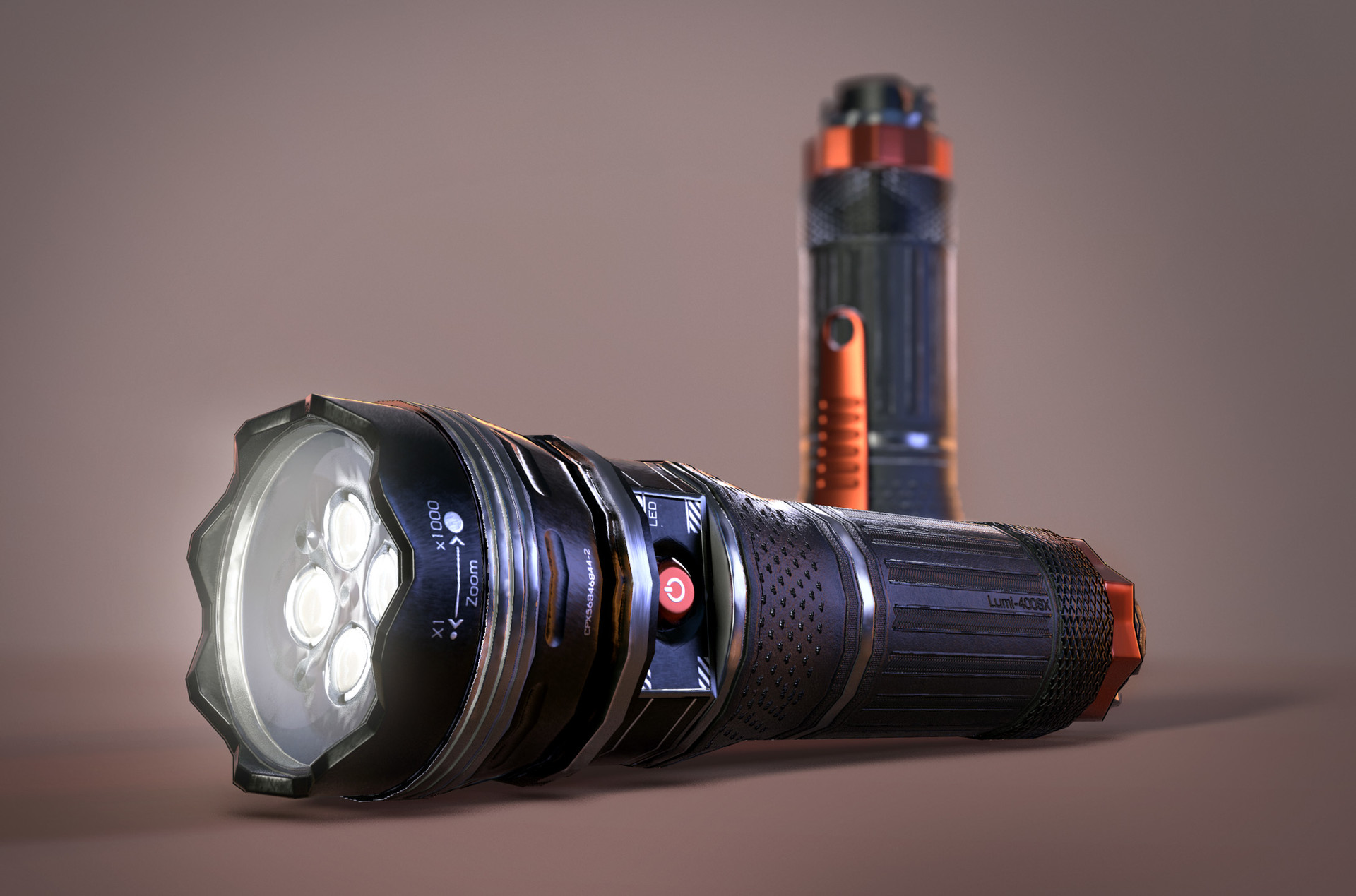The image showcases a highly detailed, 3D mock-up of two advanced flashlights, each exhibiting a sleek and modern design. The flashlights are primarily grey or black with vibrant red and orange accents. The one positioned horizontally on the ground emits a beam of light to the left, highlighting its functionality. It features a circular glass plate at the front, housing four visible bulbs. A prominent red power button is located centrally on its body. The second flashlight stands upright with its handle facing up, also adorned with similar design elements including a scalloped edge, a zoom twist, and an orange base. The flashlights appear to be part of a set, crafted with precision and likely indicative of high-end gadgets due to their sophisticated appearance. The entire scene is set against a neutral grey background, enhancing the focus on the flashlights' intricate details.